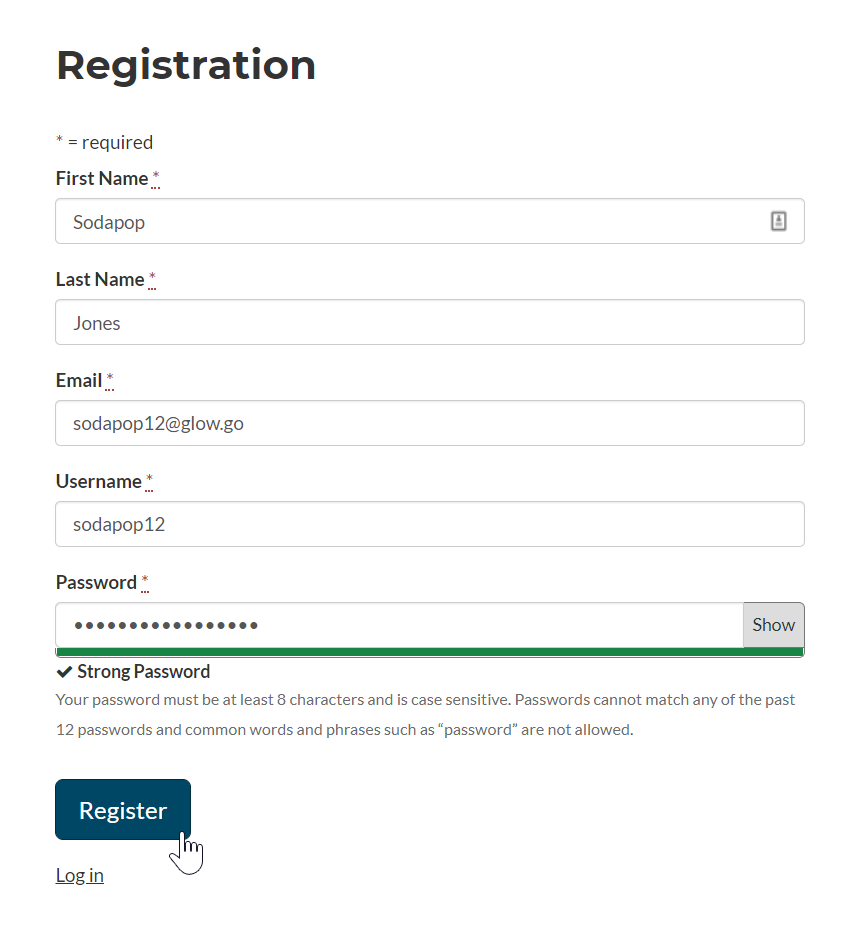This screenshot features a registration form with a white background. At the top, in bold black letters, is the word "REGISTRATION." Beneath that, in a standard font, is an asterisk followed by an equal sign and the word "required," indicating that fields marked with an asterisk are mandatory.

The form consists of several input fields:

1. **First Name**: Marked with an asterisk, indicating a required field. It contains the entry "Soda Pop."
2. **Last Name**: Also marked with an asterisk. The entry here is "Jones."
3. **Email**: Marked with an asterisk. The entry provided is "sodapop12@glow.co."
4. **Username**: Marked with an asterisk. The entered username is "sodapop12."
5. **Password**: Marked with an asterisk. The password field shows twelve black dots, indicating the entered password is obscured. To the right of this field is a gray "SHOW" button. Below the password field, the text "Strong password" is displayed with a black checkmark to its left. Further down, in gray font, it says, "Your password must be at least 8 characters and is case sensitive."

This registration form's detailed entries showcase the information provided by a user.